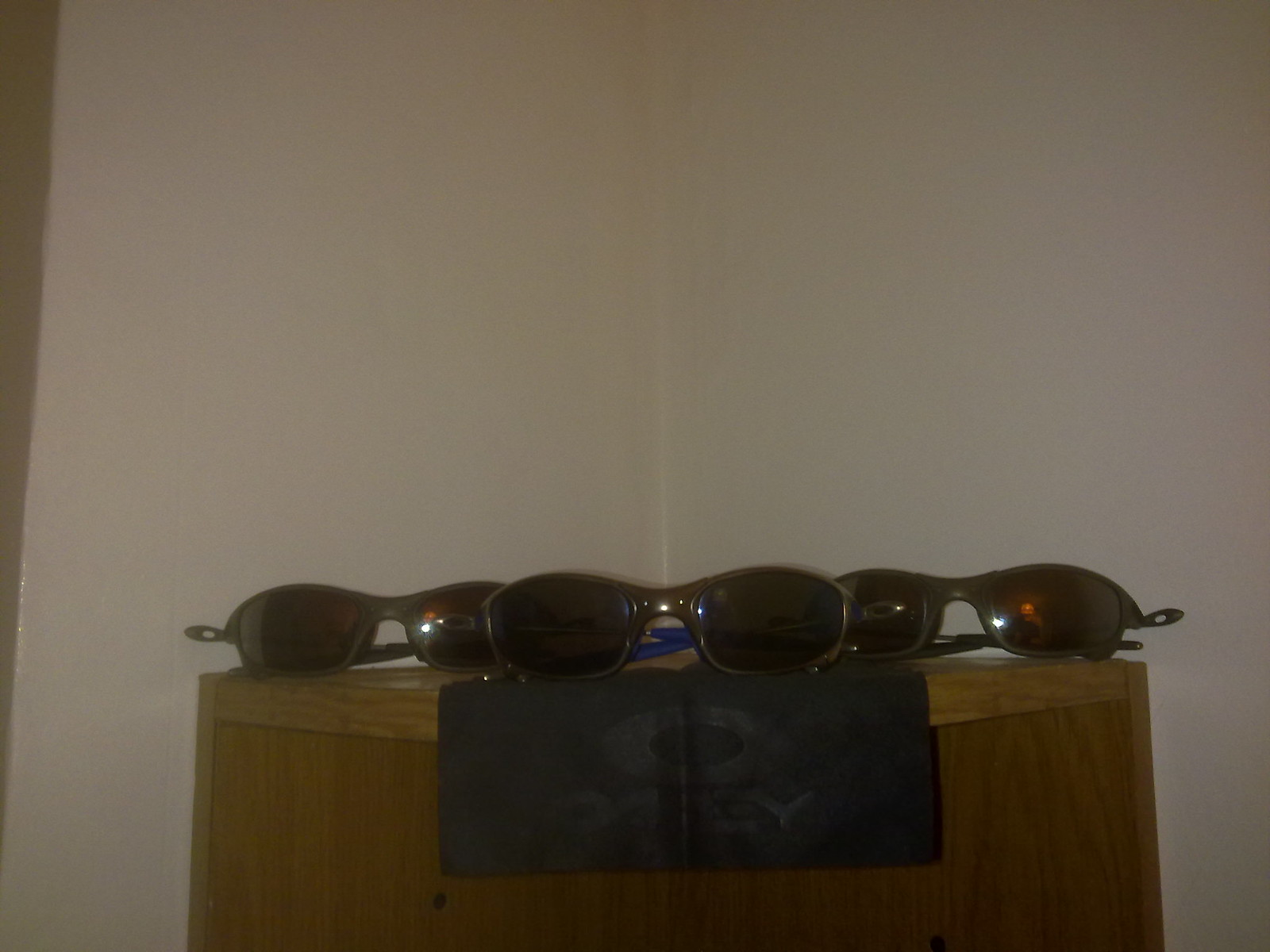This color photograph, seemingly taken indoors, features three pairs of sunglasses neatly arranged atop a dark brown wood grain box against a plain white background. Each pair of sunglasses has a similar, if not identical, style, sporting shiny metallic brown frames with dark brown or black lenses that reflect the camera flash, causing a small white starburst on the left-hand side of the lenses. The handles of some sunglasses appear darker due to the dim lighting, and there are suggestions of a red tint on certain lenses. A black fabric with a faint logo—comprised of a black oval within a white or light gray oval, and faint text reading "Oakley" beneath it—is draped over the box. The sunglasses are all positioned side by side, adding to an organized presentation. The overall dim lighting emphasizes the reflection on the lenses, hinting at the photo's indoor setting.